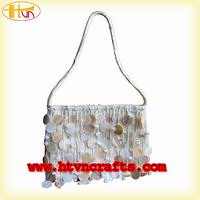This detailed image presents a small, classy evening bag prominently centered against a white background. The bag, approximately 6 inches wide and 4 inches deep, features a clasp top and a silver shoulder chain. Its body is adorned with a striking assortment of large, iridescent sequins and pearls, appearing haphazardly placed but creating an elegant and eye-catching effect with their white, cream, silver, and bronze hues on a silver backdrop.

The image also includes distinct website branding at the bottom, with the URL "www.htvncrafts.com" in bold red text. In the upper left corner, a logo is visible, consisting of an oval with the letters "HS" - where the H is yellow and the S is a reddish-auburn color, matching the oval's tone. The background of the entire image is white, softly bordered by a light yellow hue that gradually fades inward, contributing to a refined and sophisticated presentation, likely designed for a catalog or website display.